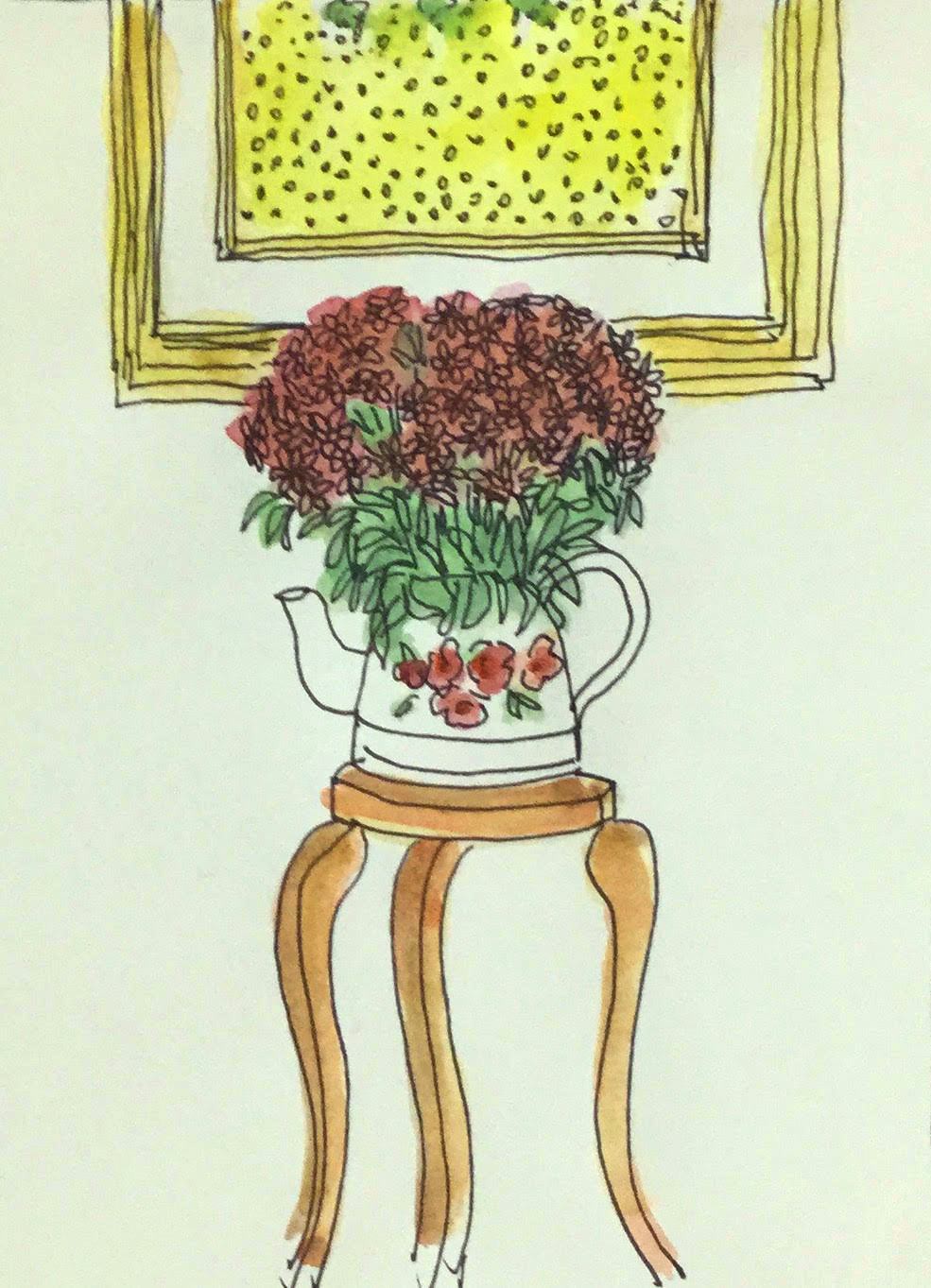This vibrant watercolor painting showcases a beautifully detailed scene set against a light green background. Central to the illustration is a slender, three-legged brown wooden table, uniquely accented with white uncolored bottom edges. Atop the table sits a white teapot-shaped vase, adorned with red floral designs. From this vase, a lush bouquet of red flowers with green stems and leaves emerges, overflowing with vivid color. In the background, a framed piece of artwork hangs on the wall. This painting features a golden yellow border that doesn't quite stay within its dark outline. Inside the frame is an intricate yellow composition with black circular dots and hints of green blotches, blending to create a brighter green hue. The artwork, anchored by a white mat, complements the scene's primary palette of yellow, brown, red, and green, tying together the minimalist yet richly detailed aesthetic.